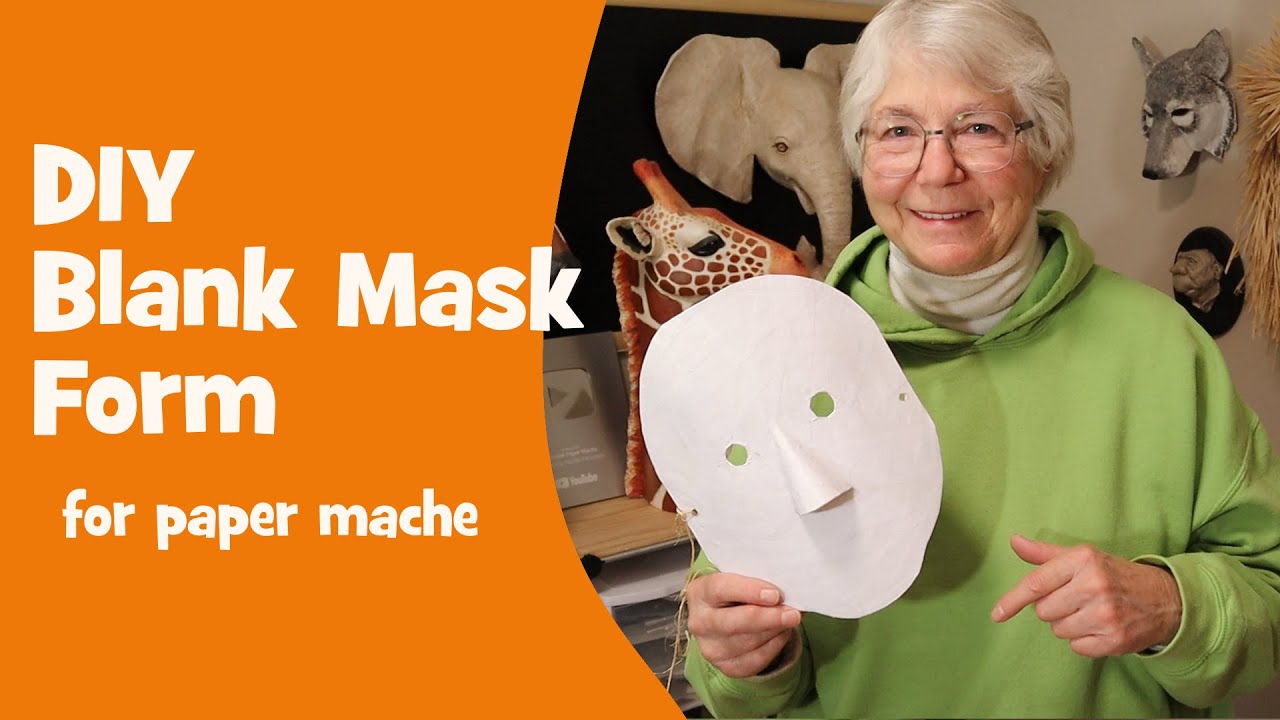The image appears to be a promotional or instructional graphic for a craft tutorial. On the left side, there's an orange, inward-curved block with bold white text declaring "DIY blank mask form" and the smaller text "for paper mache" beneath it. On the right side is a photograph of an elderly woman with fair skin, white hair, and rosy cheeks. She is wearing glasses and a green hoodie over a turtleneck. With a smile on her face, she holds a white, blank paper mask—which covers the entire face and has eye holes and a paper nose—in her right hand. Surrounding her and somewhat visible in the background are several decorative animal head busts, including an elephant, a wolf, a giraffe, and possibly a grotesque face or monkey. These elements suggest that she may be standing in a creatively decorated classroom or workshop space.